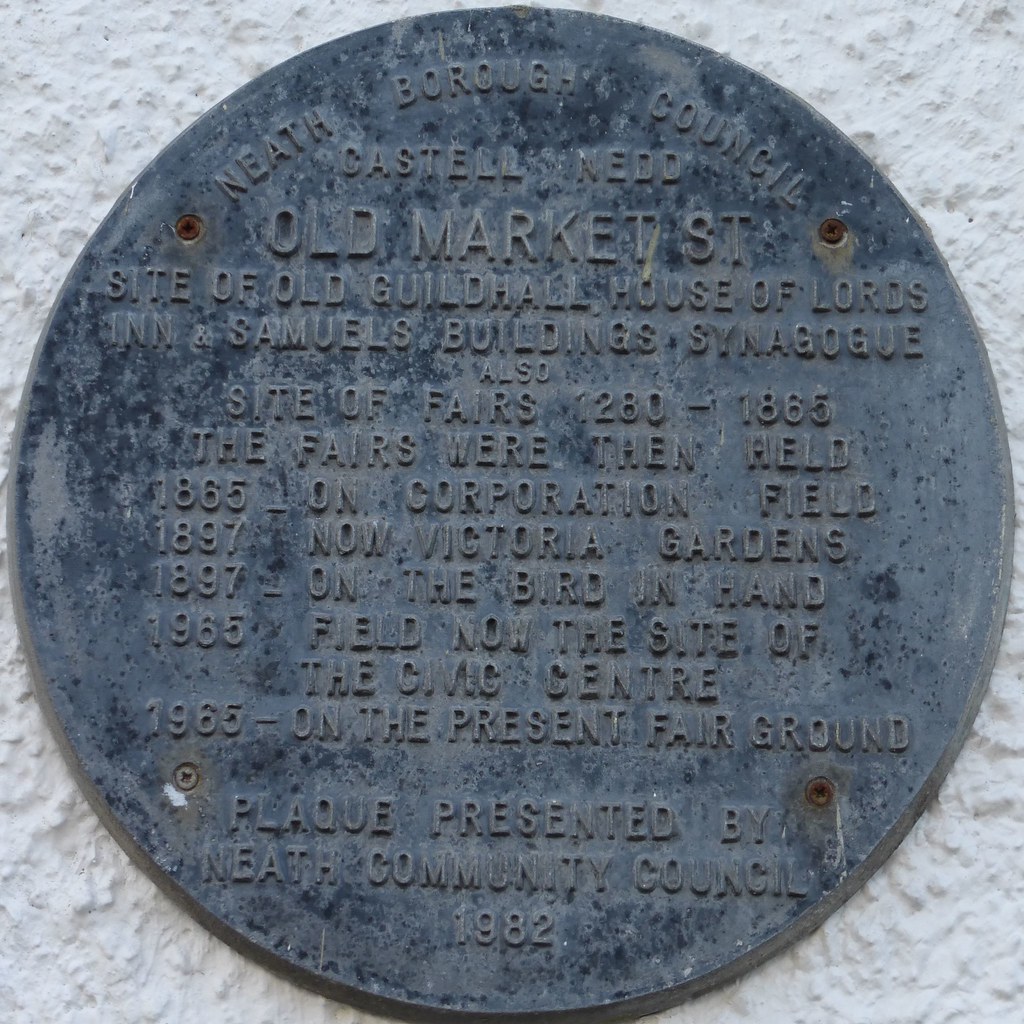This image features a close-up of a rusted, black metal plaque mounted on a white, plaster-like wall with a textured surface reminiscent of an old popcorn ceiling. The plaque, covered in heavy oxidation and displaying visible signs of age and neglect, reads: 

"Neath Borough Council, Castel Ned, Old Market Street. Site of Old Guildhall, House of Lords Inn, and Samuels Buildings Synagogue. Also site of fairs from 1280 to 1865. The fairs were then held in 1865 on Corporation Field, later Victoria Gardens in 1897, the Bird in Hand in 1897, the 1965 Field (now the site of the Civic Center), and finally on the present fairground site in 1965. Plaque presented by Neath Community Council, 1982." 

Apparent are the rusted screws securing the plaque, as well as the faded and patinaed surface, which makes the engraved text difficult to read.